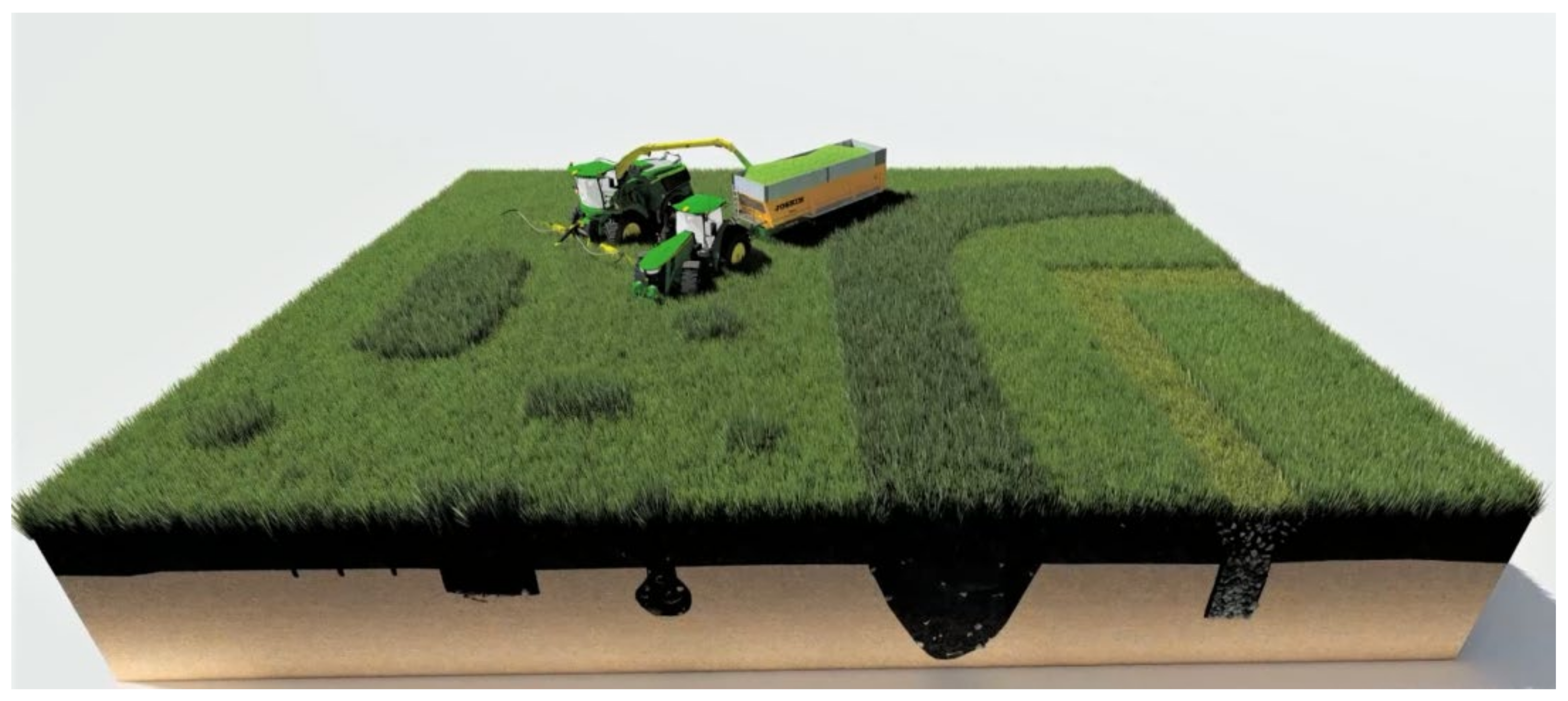This is a detailed, digitally created diagram depicting a horizontally rectangular, multi-colored image with no specific border. The background features a light blue sky. The primary subject is a green grassy field, illustrated with various shades indicating different patches and purposeful paths. In the top left, just left of center, there are three pieces of farm equipment, including a John Deere green tractor with a combine attached to a trailer, likely harvesting produce from what appears to be a cornfield. Below the verdant grass is a layer of black soil, visually representing different soil depths. At the very bottom, a shadow of an odd-looking structure can be seen. The field has sections where grass is either uncut, cut more than others, or cut into different shapes. The earthy tan beneath the green signifies the ground under the soil. The image, resembling a model rather than a live photo, also includes a base of brown wood showcasing the soil's appearance underground and the process of how grass and produce are grown. The composition of this image emphasizes the farm equipment's role in the field's distinct cutting patterns and agricultural processes.